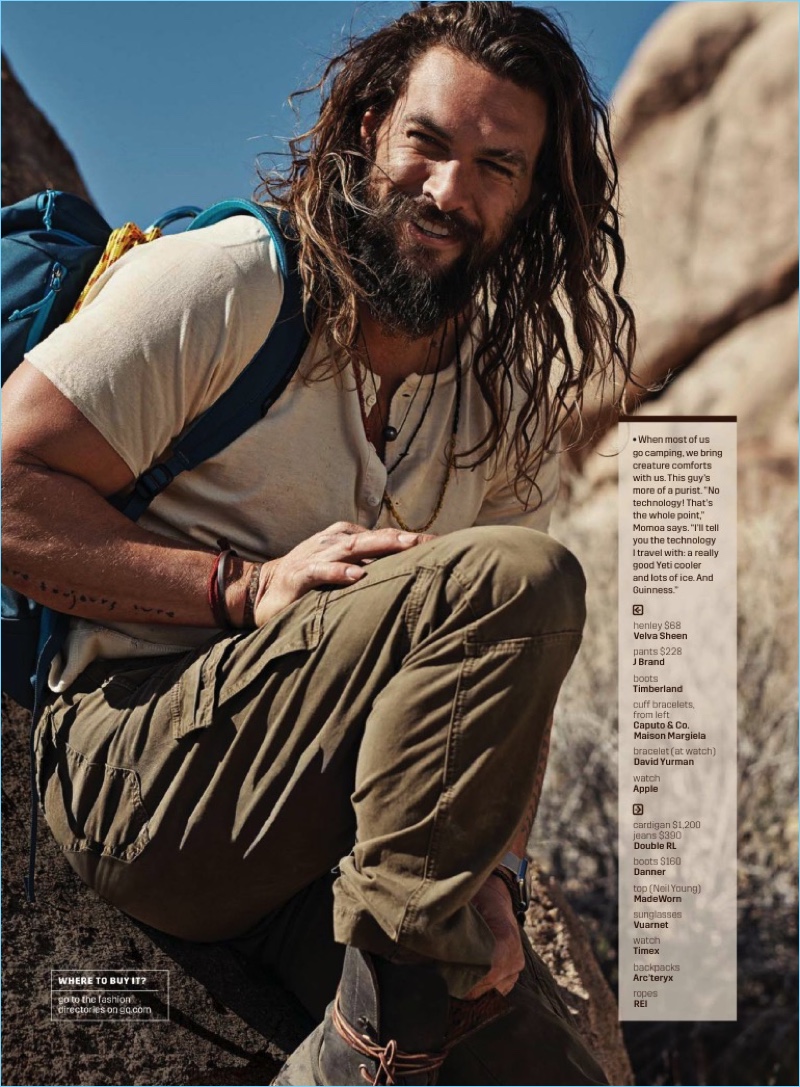In this outdoor daytime photograph, we see the actor Jason Momoa seated on the left side of a dark-colored rock. He faces towards the right but looks back slightly to the left, almost squinting as he smiles broadly, revealing his front teeth. Momoa's distinctive long, scraggly brown hair flows over his shoulders, and his full dark beard and mustache frame his face, accompanied by a noticeable scar through his left eyebrow.

Momoa is dressed stylishly yet ruggedly, donning a short-sleeved white button-up Henley shirt, olive green cargo pants, and black boots with tan and brown laces. Adorning his wrists are black and red bracelets, and he has visible tattoos on his arm and wrist. He carries a blue Arc'teryx backpack, and a yellow rope, hinting at climbing gear, is visible beside him.

To the right of Momoa, the image features a stack of lighter tan rocks with a clear blue sky above, void of any clouds. The composition of the photograph suggests an advertisement, likely a magazine spread, as indicated by the detailed descriptions along the right-hand side of the image.

The accompanying text emphasizes Momoa's minimalist approach to camping, quoting him on his preference for basic gear like a Yeti cooler, ice, and Guinness beer over high technology. It also showcases his outfit's brands and prices: a Henley Bell Machine shirt for $68, J Brand pants for $228, Timberland boots, a cardigan worth $1,200, $390 jeans, Danner boots for $160, a top by Neil Young made worn, sunglasses by Worn Up, a Timex watch, and the climbing gear by REI.

In the lower left-hand corner, the text instructs viewers to visit the Fashion Directory on GQ.com for purchasing details, underscoring the image's purpose as a fashionable lifestyle promotion featuring the charismatic Jason Momoa.